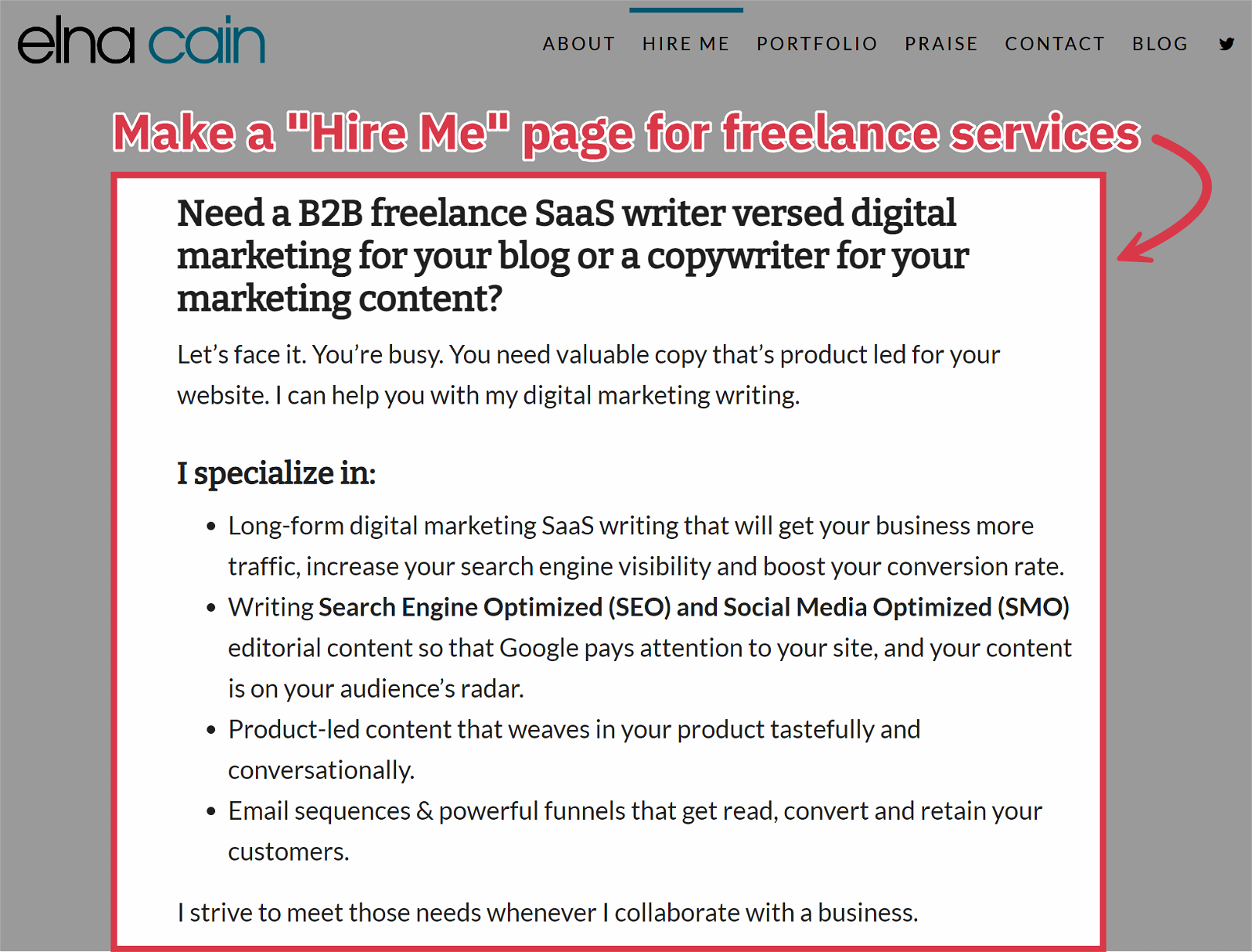In the image, there is a prominent pop-up situated in the center. The top left corner of the image displays the website name "Elna Cain," with "Elna" written in black text and "Cain" in blue text. To the right of the website name, there is a small empty space followed by several navigational categories aligned towards the top right. These categories include "About," "Hire Me" (which is emphasized by a small blue horizontal line above it), "Portfolio," "Praise," "Contact," and "Blog." Additionally, at the very top right, there is a small Twitter bird icon.

Dominating the center of the image is a square pop-up with red-toned corners. Above this square, an arrow pointing downward is accompanied by the text, "Make a Hire Me Page for Freelance Services." Inside the square, the main message reads: "Need a B2B Freelance SAAS Writer vs. Digital Marketing for Your Blog or Copywriter for Your Marketing Content." Below this, in smaller font, the text continues, "Let's face it, you're busy. You need valuable copy that's product-led for your website. I can help you with my digital marketing writing."